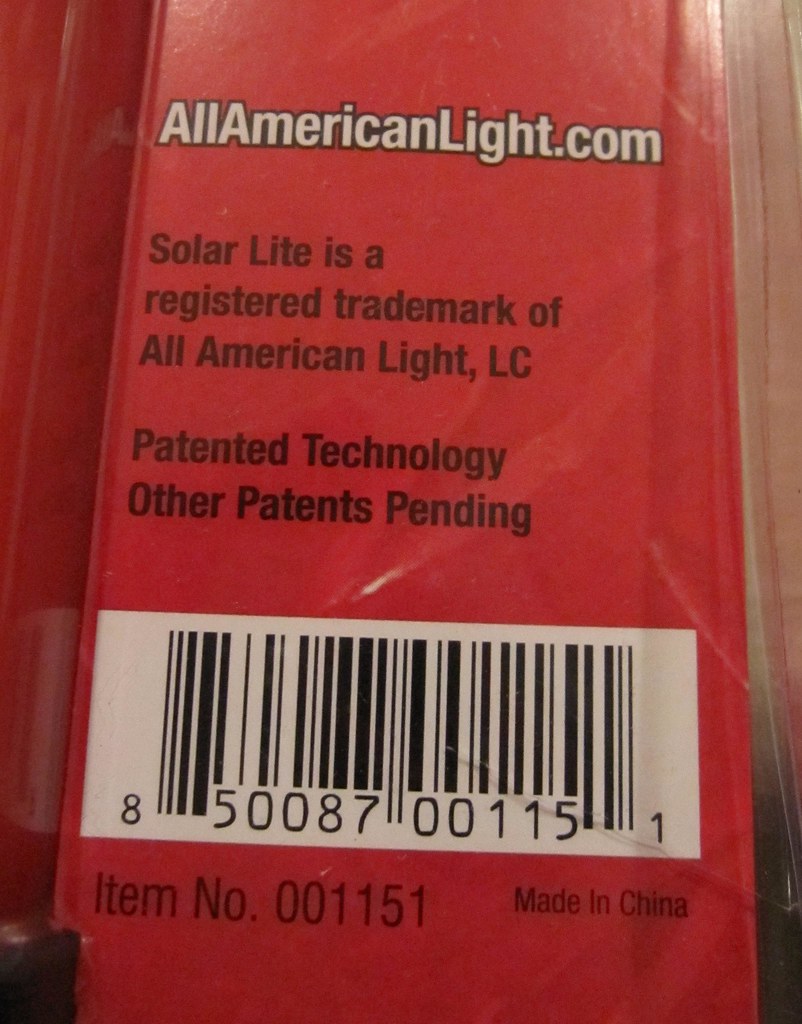The image features the text "allamericanlight.com" prominently displayed in white. Below it, the phrase "Solar Light is a registered trademark of All American Light LLC" emphasizes the brand's recognition. The statement "Patented technology, other patents pending" highlights the innovative nature of the product. At the bottom, the barcode "850087001151" is accompanied by the item number "001151". A label indicating "Made in China" specifies the product's origin. The right side of the image is filled with a brown color, providing a contrast to the informational text.